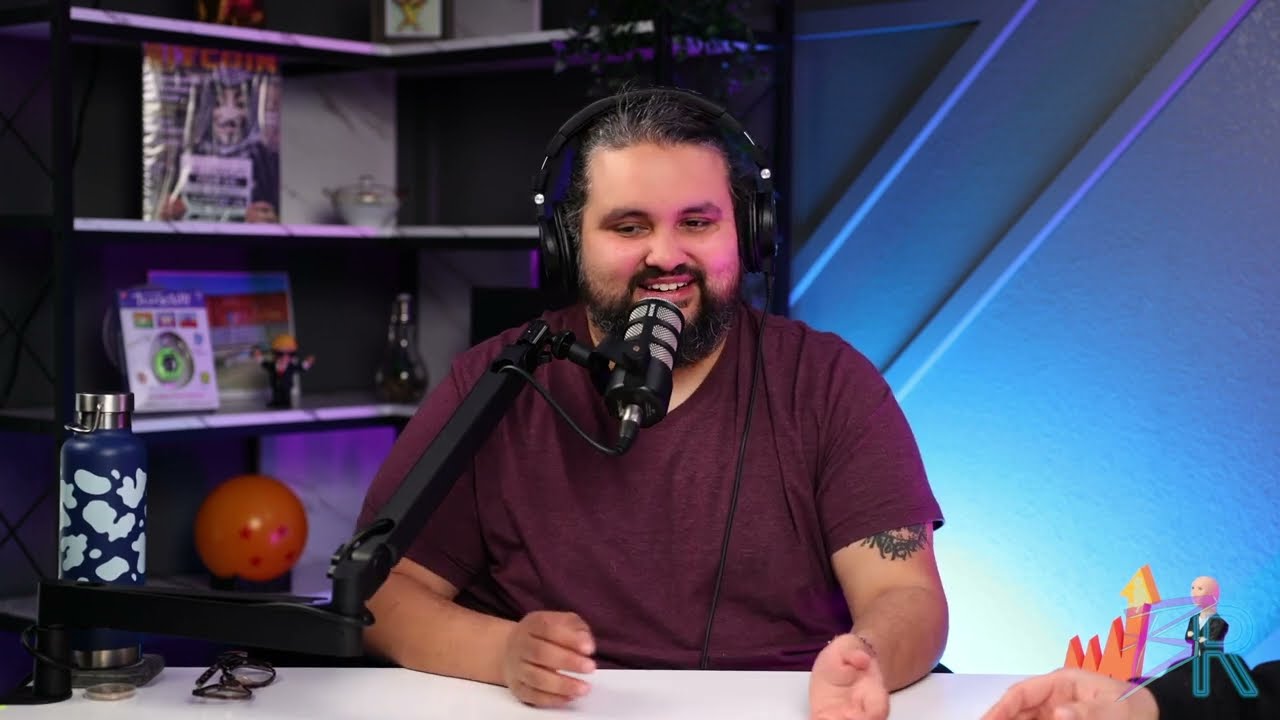This color landscape photograph depicts a podcast host seated at a white desk, engaged in a recording session. The host, a slightly overweight Caucasian man around 30 years old, sports a burgundy ring-collar shirt, a thick black and gray beard, and dark hair with streaks of gray pulled back. He wears headphones and has a microphone mounted on an arm positioned in front of him. He is smiling and gesturing with his hands, revealing a small portion of a tattoo under his right arm. 

To his immediate right on the desk, there is a dark blue water bottle with a light blue design and a pair of black eyeglasses. In the background, over his left shoulder, blue dynamic lighting illuminates a panel wall, creating a striking backdrop. Behind him, an L-shaped bookcase stretches across two walls at a corner, filled with various items, including an orange Dragon Ball from the "Dragon Ball" series, a magazine still in its cover, a model resembling the "Stonks" meme, a teapot, a vase, several books, and a vinyl record.

To the right edge of the frame, a glimpse of another person's hand and the bottom of their black shirt is visible, hinting at the presence of a co-host or guest in the podcast. The overall composition emphasizes the podcast setting enriched with personal and unique collectibles, highlighted by the vivid blue lighting that contrasts with the otherwise warm, inviting space.